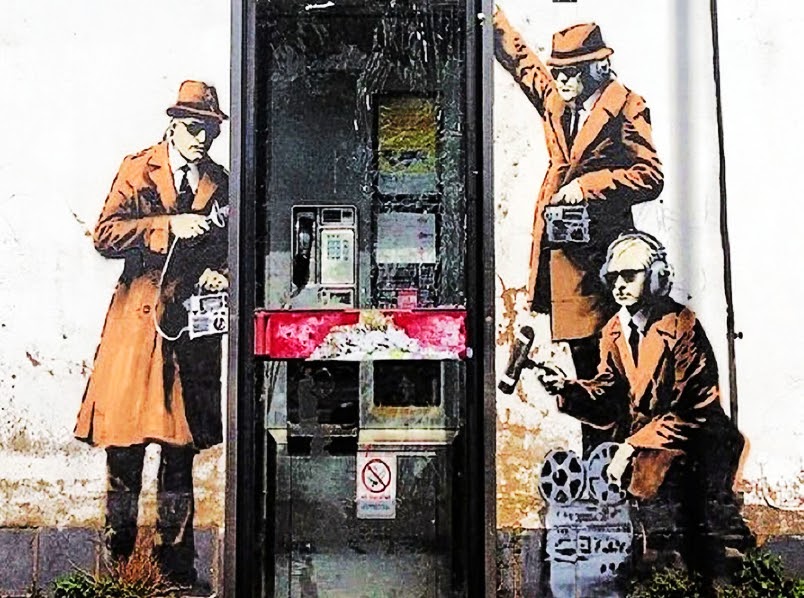The artwork features an intricately detailed, stenciled depiction of an old, worn phone booth with a red strip across its door and a dilapidated black interior, possibly reminiscent of a Banksy piece. Set against a stark white background, three men stylized as old-fashioned FBI agents in brown trench coats, fedoras, and dark sunglasses surround the phone booth, each equipped with recording devices. On the left, one man holds a radio in one hand and a microphone close to the phone booth with the other, while the man on the right mirrors this pose, also gripping a radio and clutching the top of the booth. A third man, squatting to the right, operates a reel-to-reel recorder and holds a boom microphone up to the booth, completing the surveillance scene. This silkscreen-style piece highlights themes of espionage and privacy intrusion.